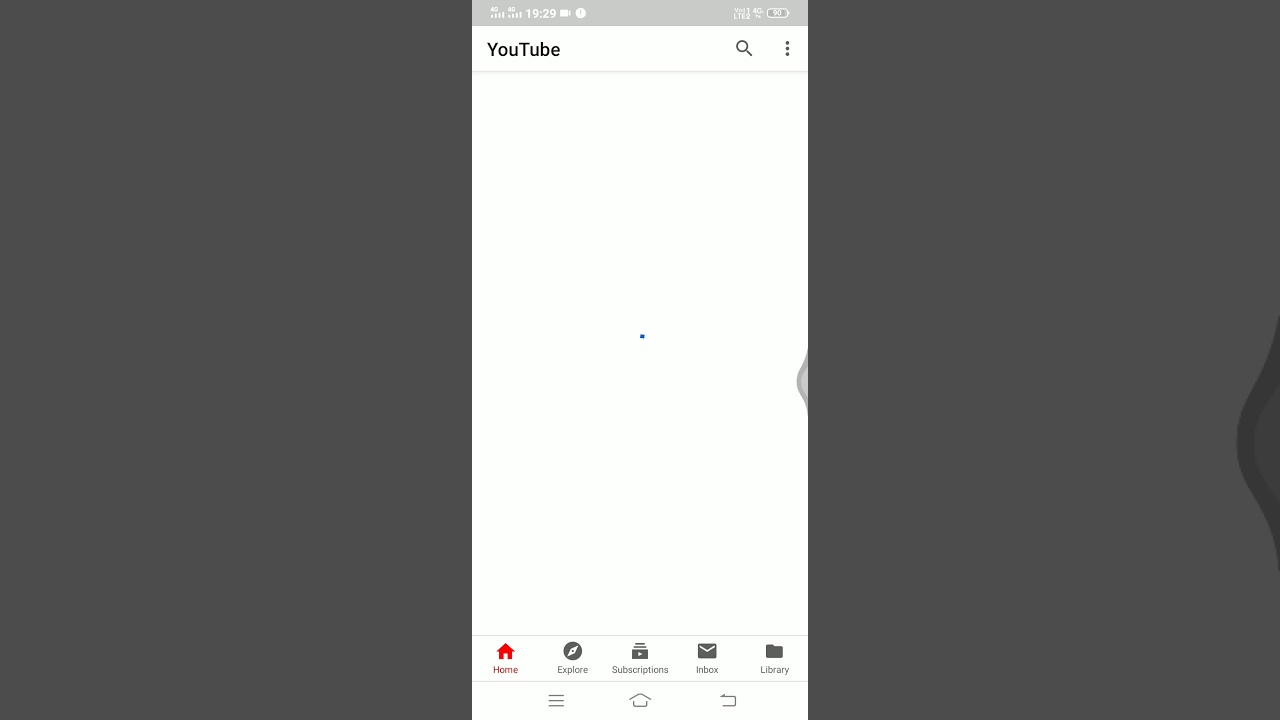The image displays a detailed screen interface of a mobile device. In the top left corner, the mobile signal strength is indicated with "4G" symbols. To the right of the signal indicators, the time is shown as "19:29" and the battery percentage reads "90%." A camera icon is also visible in this area. 

At the center of the screen, there's a black text box with a magnifying glass icon, which likely represents a search bar. Following this, there’s an ellipsis (three dots), indicating a menu option. Beneath this, a horizontal line divides the screen, with the left and right sides shaded in gray.

At the bottom of the screen, there is a red home button alongside various icons: a black button labeled "Great Accounts" for managing user accounts, an "Exports or Copies" button likely for managing files, the "Subscriptions" section for maintaining services, and "Presbyterian Book" with a box and "Library" for accessing stored content. Additionally, a "hamburger menu" icon is present, which typically opens a navigation menu.

The screen's overall layout suggests it’s part of a mobile application or operating system interface, providing various functionalities like camera accessibility, search capabilities, and user account management.